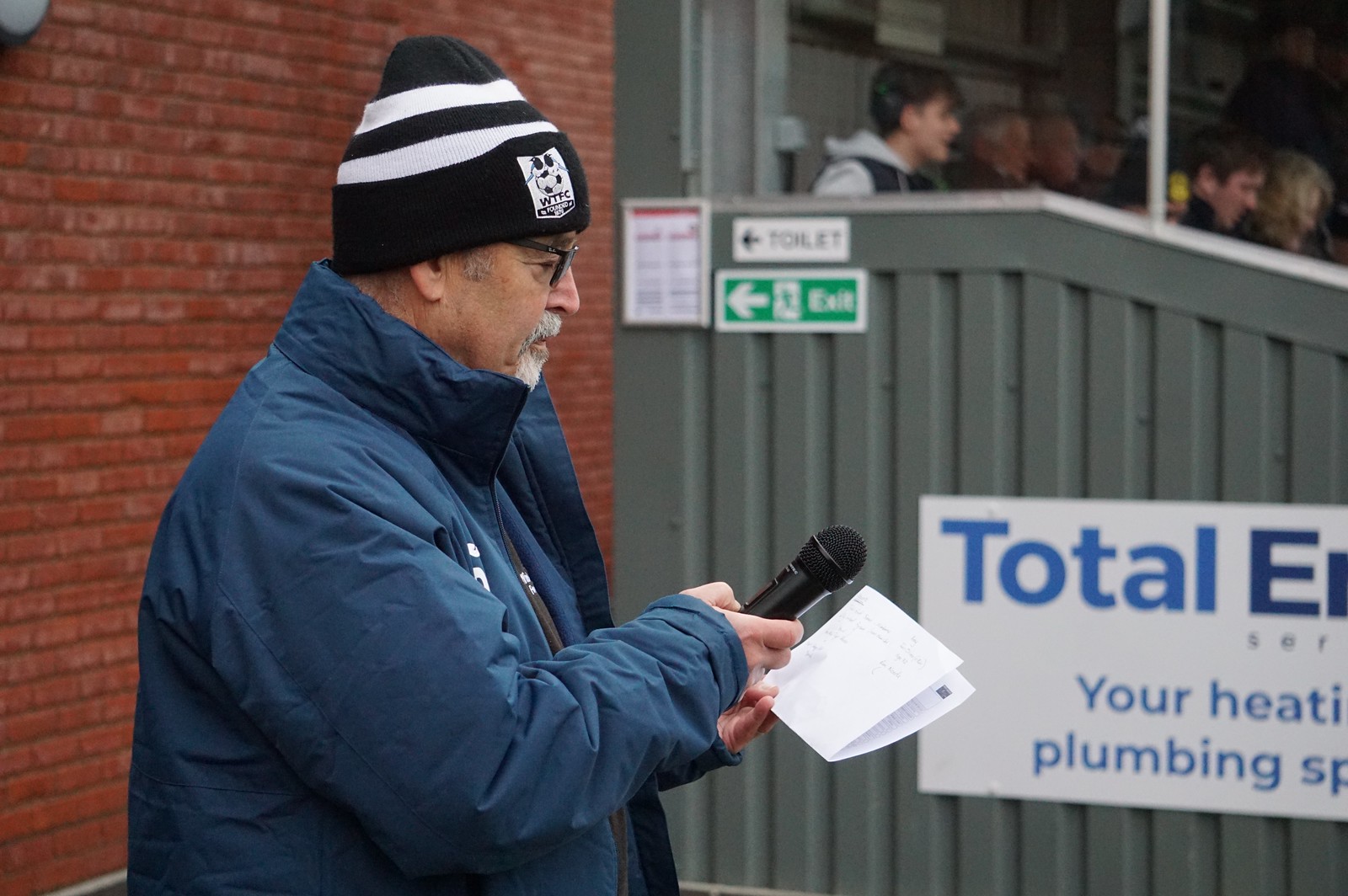This horizontally aligned rectangular photograph captures an older man from a side profile, facing right. He has gray facial hair and wears black-framed plastic glasses. On his head is a black and white striped beanie hat with a patch featuring a soccer ball and the letters "WTFC." He is dressed in an unzipped dark blue windbreaker jacket with its collar up, revealing a black sweater underneath. The man holds a black microphone in his right hand and a folded sheet of paper in his left, which he is looking down at, suggesting he may be preparing to give a speech or presentation.

In the background, the left side features a red brick wall with multiple signs indicating the locations of a toilet and an exit, both with leftward arrows. Adjacent to him on the right side is a gray corrugated steel wall with blue-lettered signage, partially visible, reading "total E." Further to the right, there appears to be a small stadium seating area with some people seated, possibly on benches. This setting suggests an outdoor venue, adding to the overall context of the image.